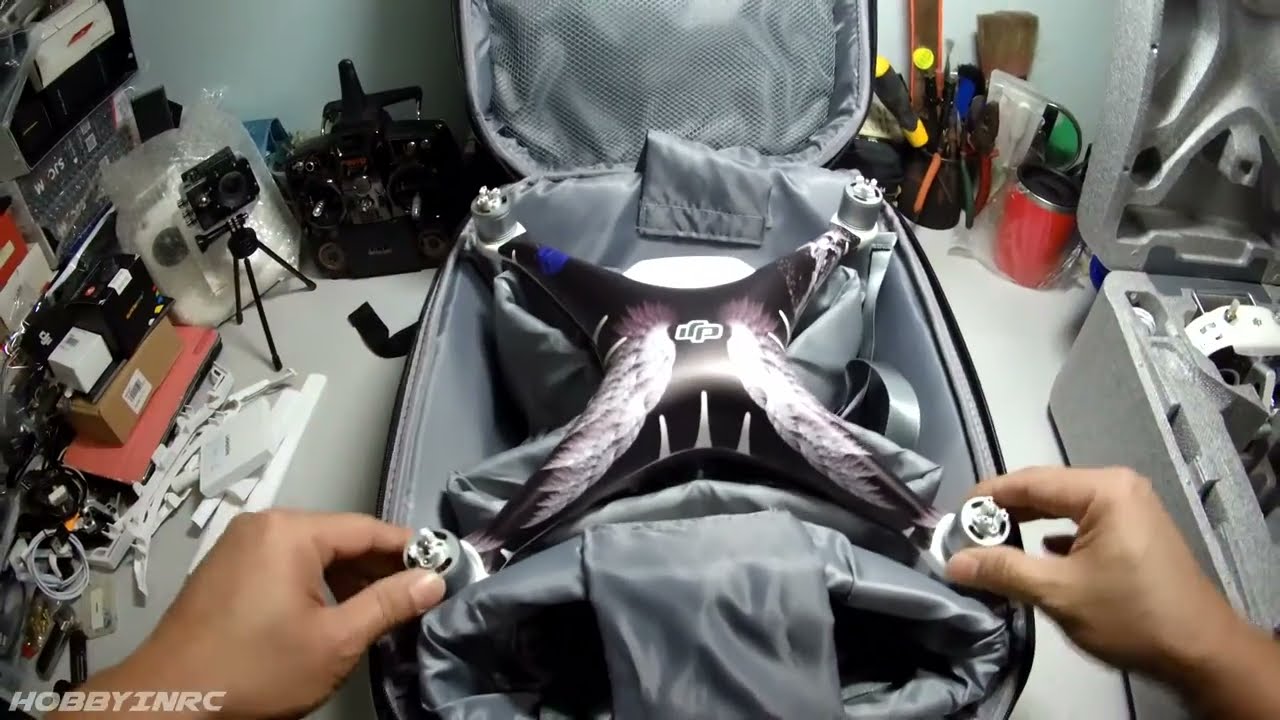The image depicts a person manipulating a star-shaped device with four sides, securely strapped inside an open, gray-interior carrying case. The device, likely a tripod or a related accessory, is held by tan human hands operating two controllers placed on a pillow within the case. Surrounding the case are various tools, including screwdrivers, other utensils, and several cups. There are also camera features and accessories scattered around. In the background, a black camera mounted on a tripod stands against a predominantly gray workspace, cluttered with small electronic parts, boxes, and additional accessories. This area is further highlighted by a lime-green wall behind the setup.